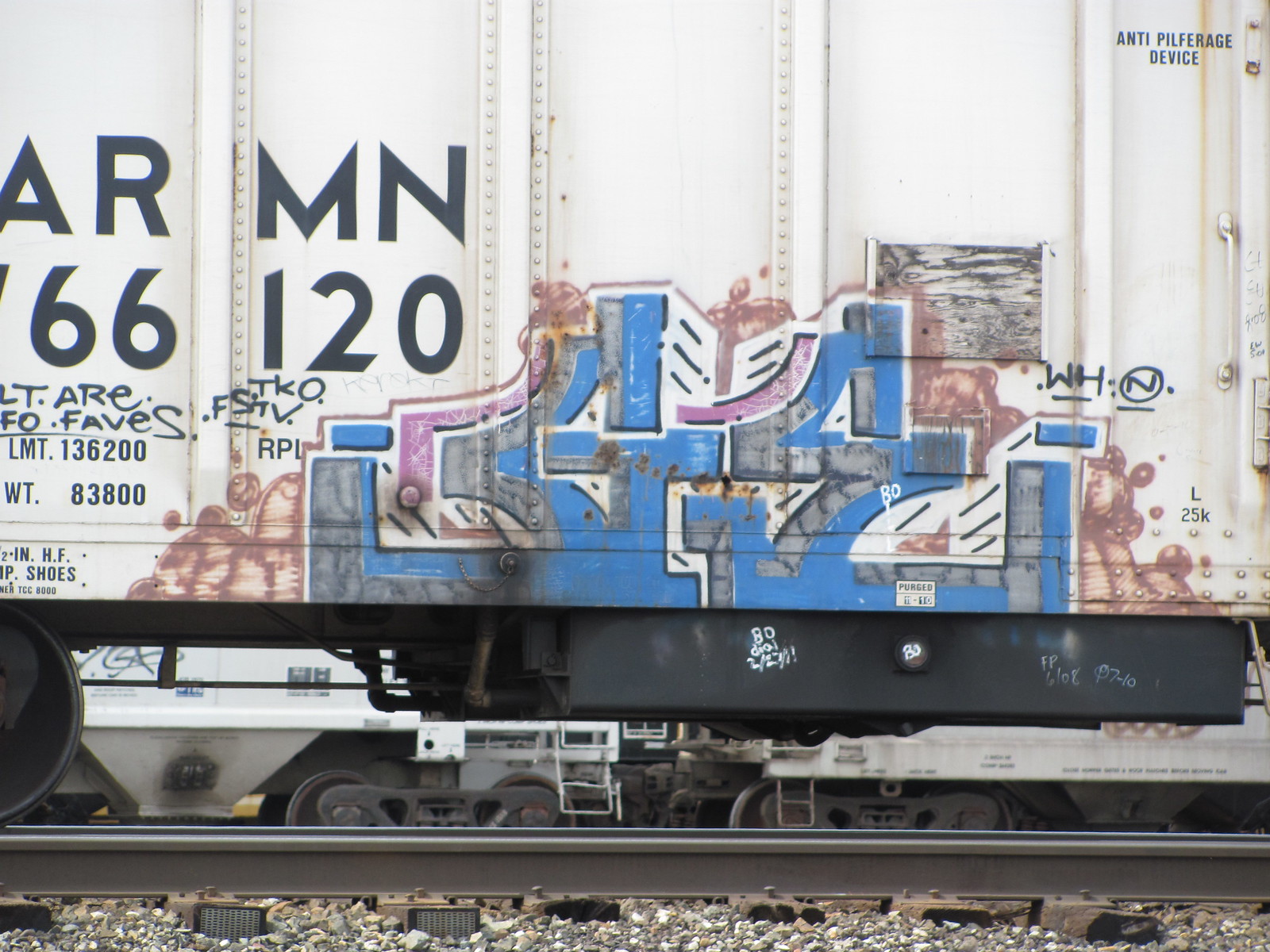The image depicts a detailed side view of a weathered, whitish-grey cargo boxcar positioned on train tracks with a mixture of white and black pebbles beneath. The tracks feature dark grey steel rails and wooden ties. The boxcar, marked with rust and graffiti, bears substantial black lettering that reads "AR MN 66120" on the left side. Below this text, it states "LMT.136200" and "WT.83800" in black letters. Towards the center of the boxcar, prominently visible is blue and pink graffiti, possibly foreign or consisting of symbols, with interpretations ranging to suggest it could denote the number "44". Further down on the black undercarriage, smaller white graffiti is evident. On the top right corner, there is a small, clear black text indicating an "Anti-Pilferage Device". In the background, additional boxcar wheels and another train or locomotive can be seen, suggesting multiple tracks.